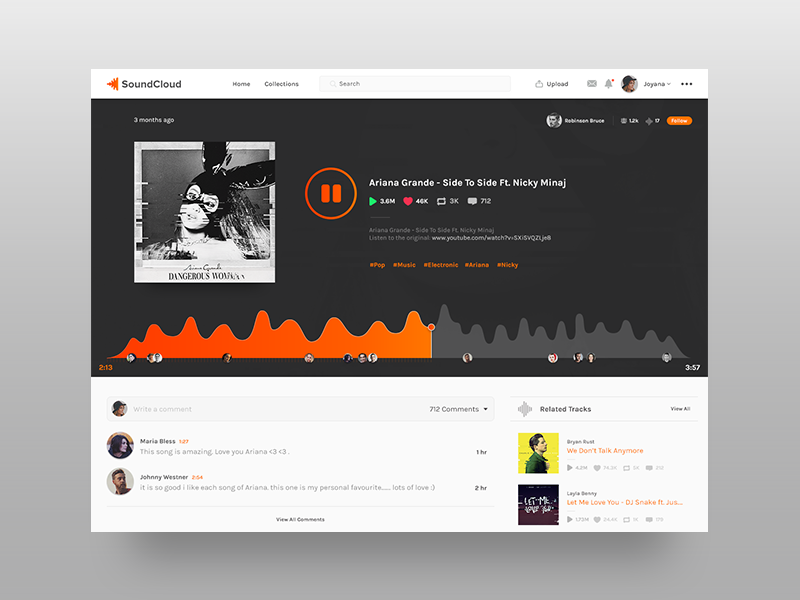The image is a detailed screenshot of a SoundCloud page. The interface is framed by a thick gray border with the actual content centered. At the top of the page, a white bar prominently displays the SoundCloud logo alongside navigation options like Home, Collections, a search bar, and an Upload button. The user appears to be named Joyanna, indicated by the profile name "JOYANA" and a thumbnail photo depicting a woman in a black hat looking off to the right.

Beneath this header is a large, visually-striking, black-and-white Polaroid-style photograph featuring Ariana Grande in a black cap adorned with bunny ears. This image is captioned "Ariana Grande - Dangerous Woman." To the right of the photograph, there is a large orange play button.

Below this primary image, we're given details about the track "Side to Side" featuring Nicki Minaj. The song has been played 3.6 million times, garnered 46,000 likes, 3,000 replays, and 712 comments. The track is categorized under several hashtags such as #pop, #music, #electronic, #Ariana, and #Nicki. Additionally, a waveform visual representation of the track is visible, with the left section of the wave colored in orange and the right side in gray.

Two prominent comments are displayed beneath the waveform. Melissa Bless writes, "This song is amazing. I love you, Ariana." Johnny Westner adds, "It is so good. I like each song of Ariana. This one is my personal favorite. Lots of love."